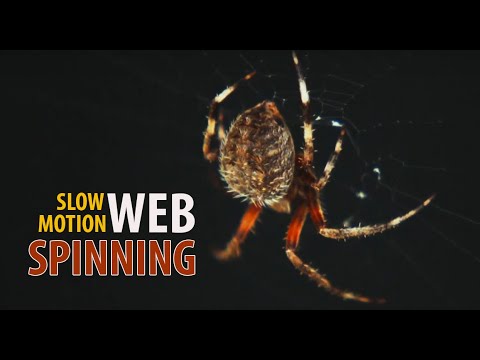This close-up photograph captures a large brown spider with distinct teardrop-shaped body and legs adorned with alternating blotches of black, white, and red. The spider is positioned on the right-hand side of the image, seemingly in the act of spinning a web. The background is entirely black, enhancing the spider's detailed appearance. On the lower left-hand side of the image, text in various colors reads “Slow Motion Web Spinning,” with "Slow Motion" in yellow, "WEB" in large white uppercase letters, and "Spinning" in reddish brown with a white outline. The overall dark atmosphere accentuates the intricate details of the spider and the text.